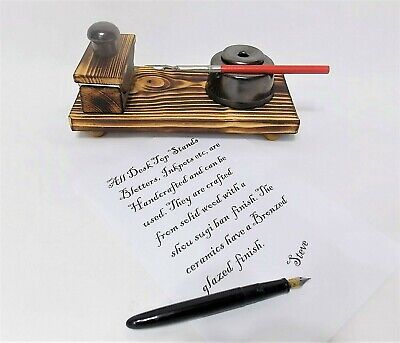This image features an advertisement showcasing artisanal desk items. In the center at the bottom of the image is an elegant, thick black pen with a golden tip. Above the pen, there's a piece of handwritten text, presented diagonally and somewhat difficult to read due to its small, stylized font. The text reads, "All desktop stands, blotters, ink pots, etc. are handcrafted and can be used. They are crafted from solid wood with a shōsugi-ban finish. The ceramics have a bronze-glazed finish," and it is signed "Steve."

At the top of the image, there's a meticulously detailed drawing or possibly a photograph of a desk setup. This setup includes a wooden calligraphy stand with a shiny black handle attached to a wooden piece, resting on two wooden legs. Adjacent to the stand, there's a black cylindrical inkpot with two smaller black shapes—a cylinder and a sphere—on top of it. Positioned on this inkpot is a utensil that seems to be a paintbrush or a fancy pen with a red handle and a steel tip.

The background of the image is plain white or gray, enhancing the focus on the intricately designed and finely finished wooden and ceramic desk items, underscoring their handcrafted quality and stylish presentation.